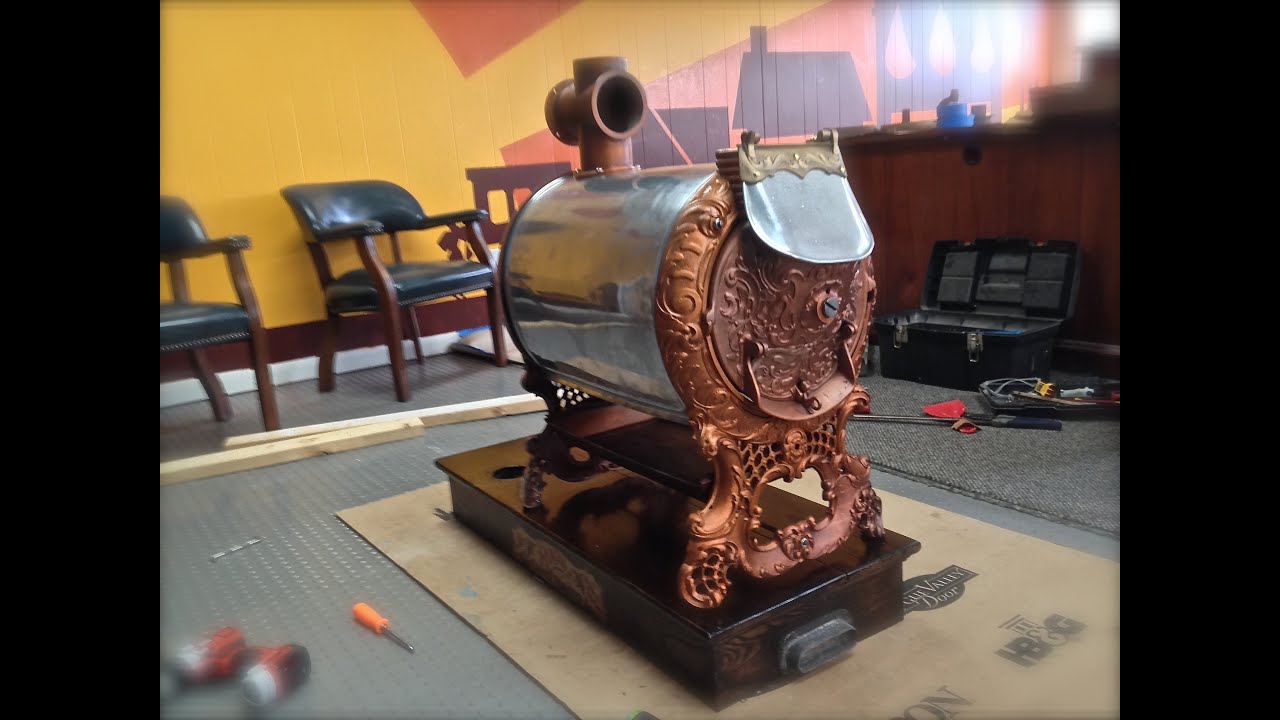The photograph depicts a vintage cylindrical device, potentially a coffee roaster or water heater, positioned horizontally on a wooden platform. This cylindrical unit is made from a silver, possibly stainless steel, material and is supported by intricately designed, copper or bronze-colored metal supports. The entire assembly rests on a tan mat that covers the floor beneath it. Surrounding the base are scattered tools including an orange screwdriver and a red electric battery-operated drill, indicating ongoing work. 

In the background, an open toolbox further suggests maintenance or repair work being conducted. The setting includes a yellow wall and two leather upholstered chairs with wooden legs. The image exhibits a slightly blurred vignette effect around the edges, emulating a Barbara Walters-style soft focus, while maintaining crystal clarity in the center. The scene is brightly illuminated, emphasizing the blend of vintage craftsmanship and the contemporary workshop setting.